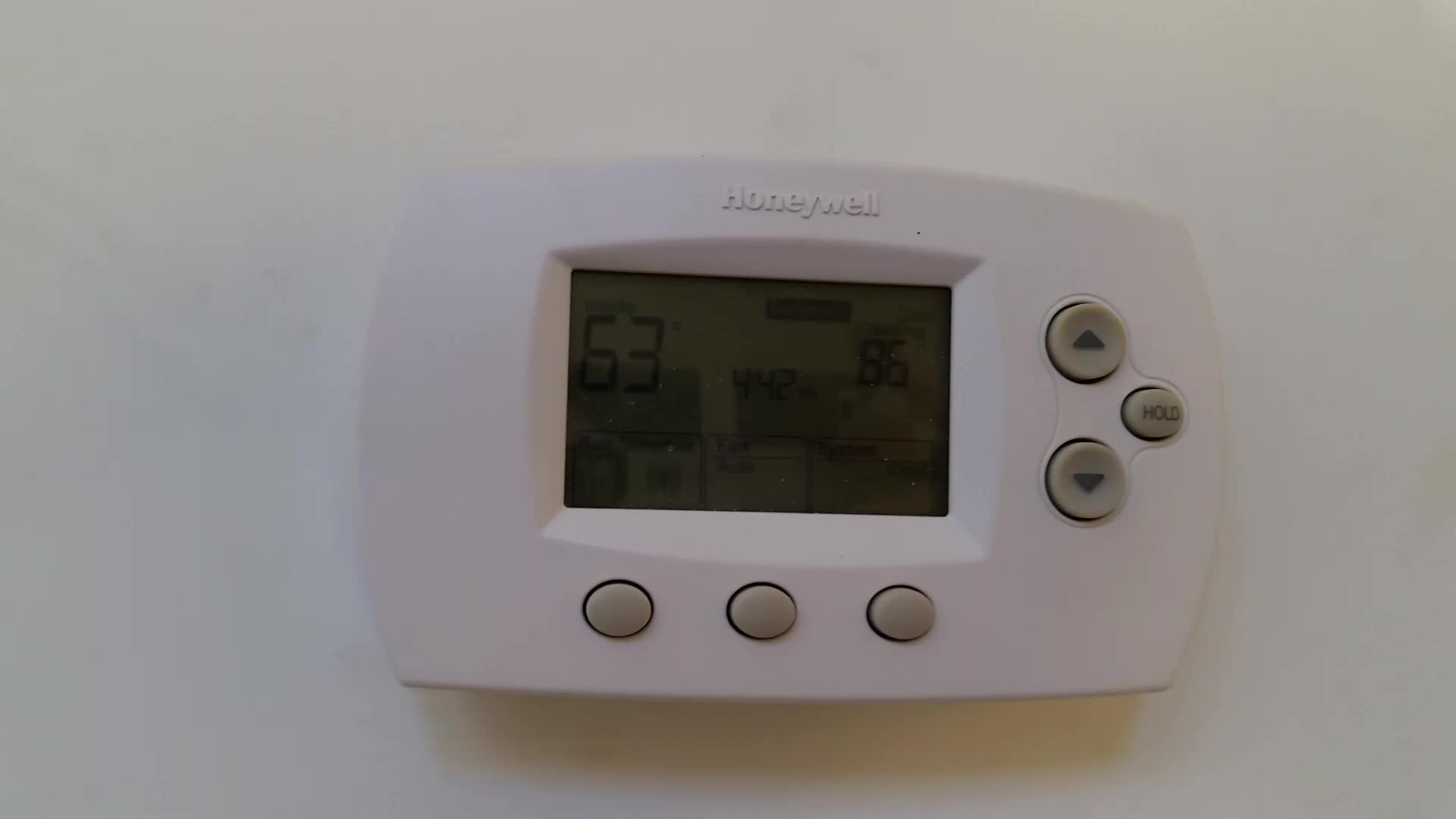A detailed caption for the image could be:

"This digital thermostat display, manufactured by Honeywell, features a modern, functional design. Encased in a white plate, the thermostat includes multiple control options. The centerpiece is a grayscale LCD display that shows essential information including the current temperature (set at 63 degrees), the date and time, the operational mode, the day of the week, and fan status. Along the bottom, there are three selection buttons for navigating the screen's menus. On the right side, adjacent to the directional up and down buttons for temperature adjustment, is a dedicated 'Hold' button for maintaining settings. The thermostat is mounted on a clean, white wall, and a slight shadow falls across the device, adding depth to the image."